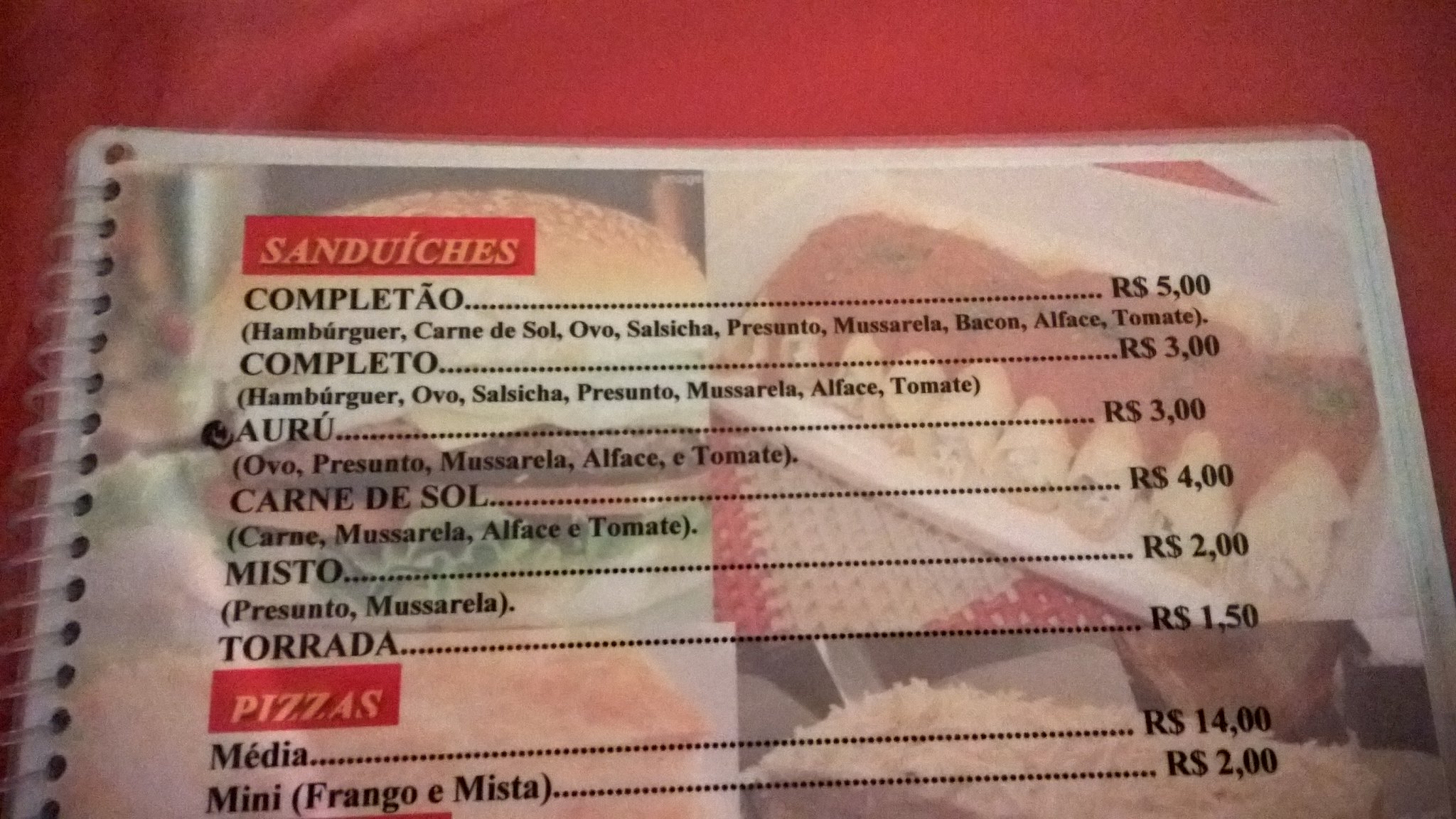This photograph features a slightly grainy, landscape-oriented image of a restaurant menu placed on a red fabric tablecloth. The menu, which appears to be a spiral-bound notebook with printed, possibly laminated pages, displays text in a foreign language that might be Portuguese or Spanish. The top of the menu prominently features the word "SANDUÍCHES," suggesting a section dedicated to sandwiches. Faded background images depict a burger and what seems to be a pasta dish, adding a visual context to the offerings. The menu lists various dishes with their ingredients alongside prices, marked in a currency denoted by the letter 'R' and a dollar symbol, with amounts ranging from 1.50 to 5.00. The bottom part of the menu mentions "PIZZA," indicating another category of food items available.